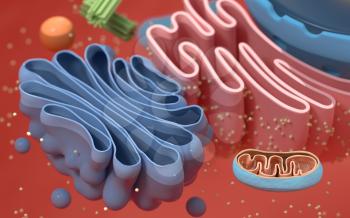This detailed sculptural illustration showcases a vibrant assortment of intertwined ribbons and various shapes set against a reddish-pink background. Predominantly, there are two main ribbons: a blue ribbon with several folds positioned on the lower left and a pink ribbon adorned with intricate swirls to its right. Below these ribbons, a cluster of blue balls and one prominent brown ball are featured. The lower right corner reveals a lighter blue ribbon that encapsulates another coiled ribbon within its embrace. 

In the upper part of the image, there is a green tubular device emerging from the upper left, wrapped in green material, suggesting a possible structural or connective role. Additionally, the upper right contains a blue container, which seems to hold more ribbons, contributing to the layered and complex arrangement.

The imagery bears a certain anatomical resemblance, with shapes suggestive of human internal parts. The blue ribbon and the pink ribbon lay next to each other, unraveled, drawing the viewer's eye toward their sinuous paths. Floating around the composition are numerous small tan-colored balls, three medium-sized blue balls, and a slightly larger orange ball. Completing this eclectic mix are two green stalks resembling celery, positioned at the top, adding an organic touch to this intricate, ribbon-filled tableau.